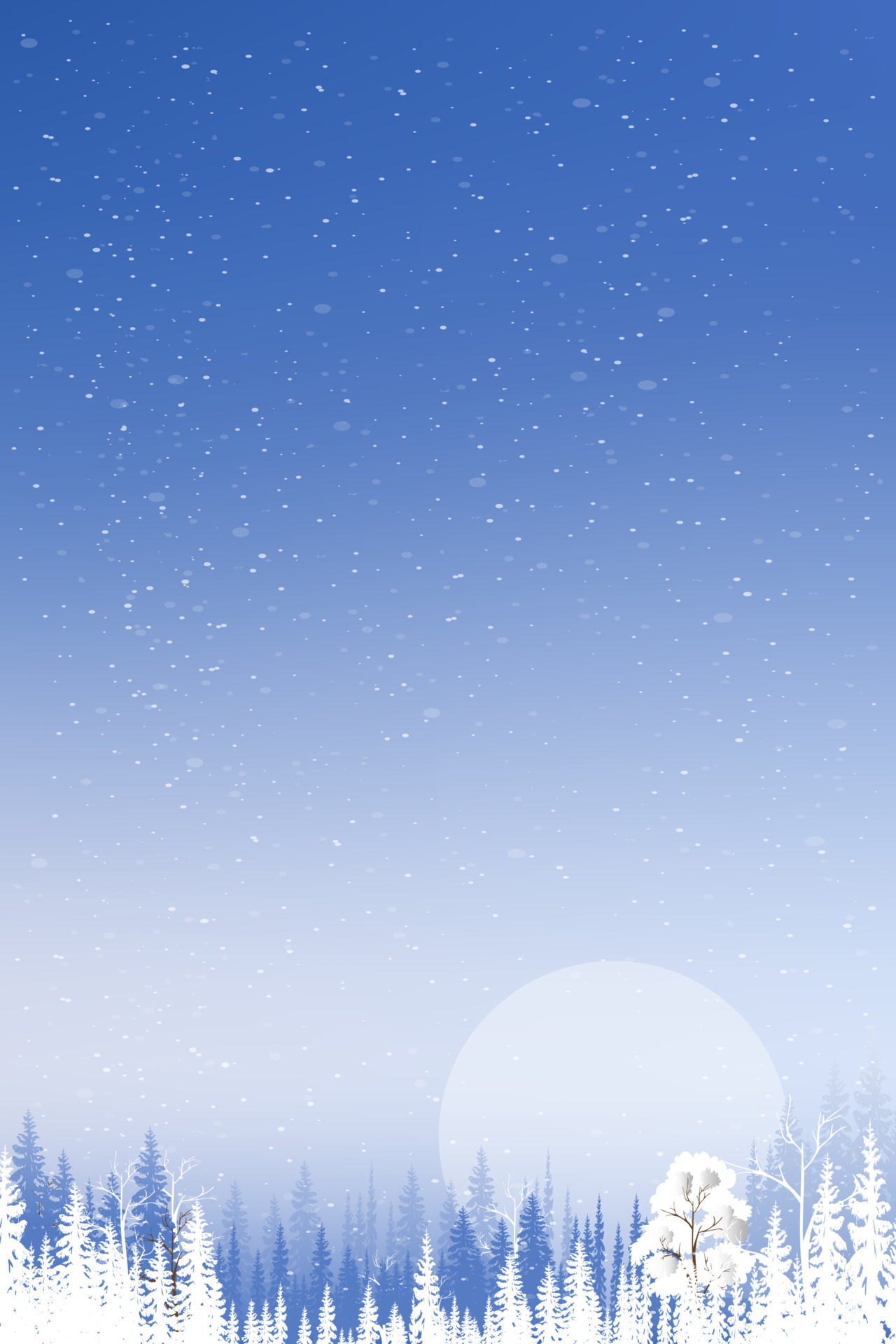This artwork depicts a serene winter landscape during twilight, dominated by a striking sky. At the top, the sky is a bright, bold blue which gradually transitions to a near-white hue as it meets the horizon, creating a vivid ombre effect. Scattered across the sky are white specks, representing delicate falling snow. On the right side, there's a prominent, tall tree distinct from the evergreens, detailed with bark and branches, its leaves heavily coated in snow, giving a pristine, white appearance. The ground is depicted in pure white, simulating a thick blanket of snow. The lower portion of the image showcases three distinct rows of evergreen trees, their colors ranging from white in the foreground to darker and more muted shades of blue and gray in the background, enhancing the sense of depth. Near the horizon, a large, round, solid white circle – potentially the sun or moon – rises, casting a serene glow over the tranquil winter scene.